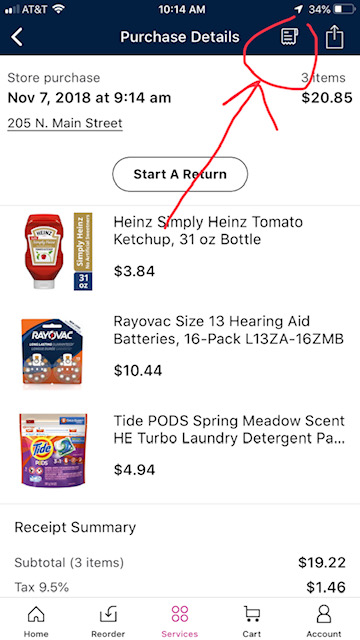The image showcases a cell phone screen displaying a detailed purchase receipt with several UI elements visible. On the left side of the status bar, there are signal bars indicating cell service from AT&T, and bars indicating Wi-Fi connection strength are displayed in the center. The current time, "10:14 AM," is centered in the top bar, while the battery life shows 34% on the right. The entire screen is set against a black background.

Below the status bar, there is a back arrow labeled "Purchase Details" and an icon of a receipt, circled in red using a photo editor tool. An arrow, also drawn in the image, points to the receipt icon from a specific item, indicating a "Starter Return" process. 

The detailed items listed are:
1. Heinz Simply Heinz Tomato Ketchup, 31 oz bottle priced at $3.84 (highlighted by the arrow pointing to the receipt icon).
2. Rayovac Size 13 Hearing Aid Batteries, 16-pack (L13ZA-16ZMB), priced at $10.44.
3. Tide Pods Spring Meadow Scent HE Turbo Laundry Detergent, priced at $4.94.

The receipt summary includes:
- Subtotal for the three items: $19.22
- Tax: $1.46
- Total after tax: $20.68

At the bottom of the screen, there are options for "Home," "Record," "Services," "Cart," and "Account," separated by a line from the receipt details.